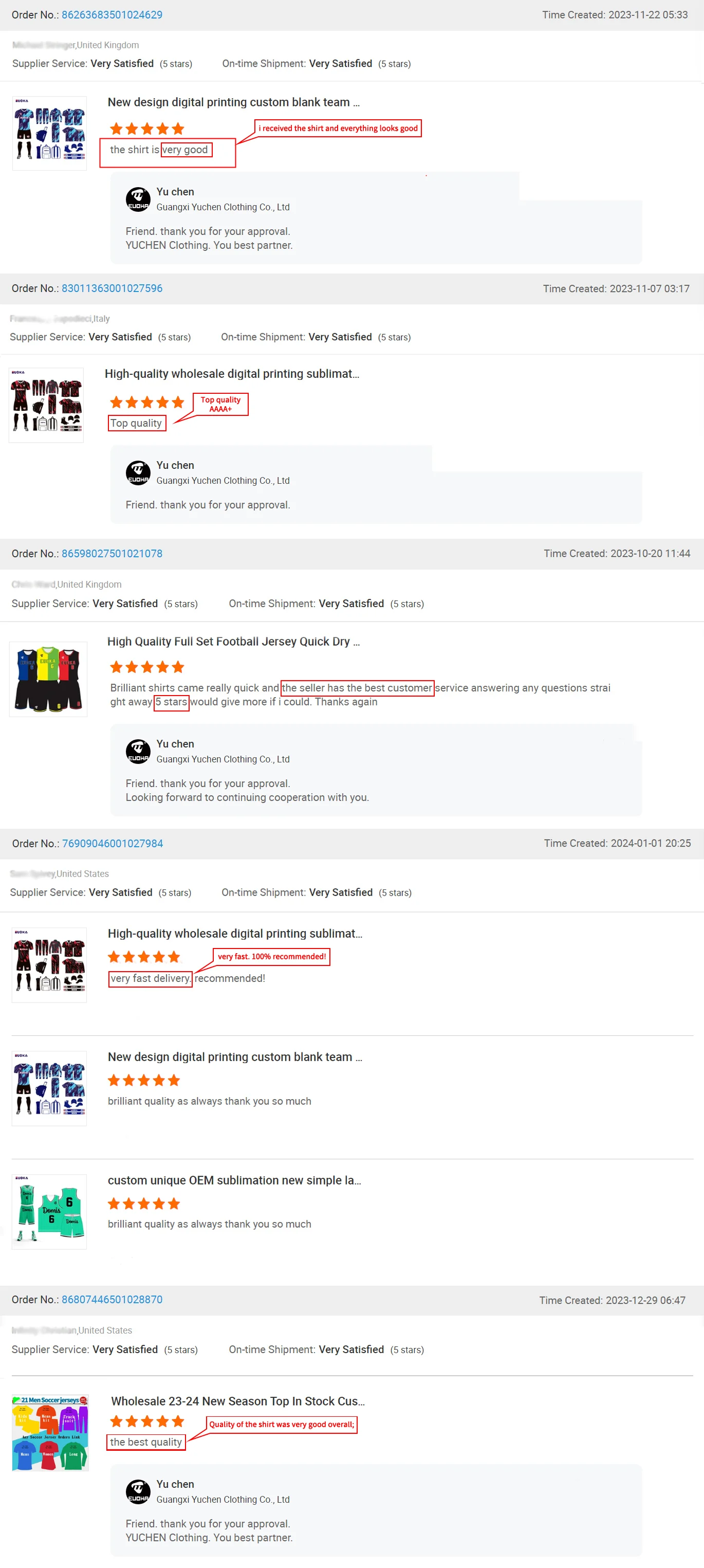The image shows an overview of various order numbers from a supplier, highlighting customer satisfaction. At the very top, order number 862-636-83501024629 is displayed in blue, accompanied by ratings of "Supplier Service: Very Satisfied, 5 stars" and "On-Time Shipment: Very Satisfied, 5 stars." The customer praised the shirts they received, describing them as very good. The response from the supplier, You Chin Clothing, reads, "Friend, thank you for your approval. You Chin Clothing, your best partner." This particular order was created on November 22, 2023.

Another order, created on November 7, 2023, features similar clothing items, mainly shirts, and was rated "Top Quality: Very Satisfied, 5 stars" and "On-Time Shipment: Very Satisfied, 5 stars." The supplier once again thanked the customer for their approval.

Overall, the image showcases multiple orders of sportswear, particularly for different sports teams, all receiving top ratings and displaying blocked-off sections that hint at the seller's excellent reputation. The consistent 5-star ratings and comments such as "100% recommended" and "Very fast delivery" emphasize the high level of customer satisfaction with You Chin Clothing.